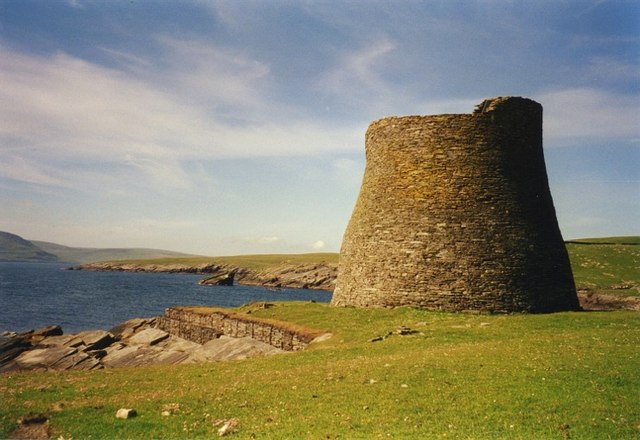The landscape image showcases a serene and captivating outdoor scene dominated by an ancient, cylindrical stone structure, possibly a ruin of an old tower. This structure, which appears to be constructed from gray and brown stones, stands on a field of green grass tinted with patches of yellow. To the left of the tower, there is a hand-carved ledge with manmade rock slabs, hinting at human intervention in shaping the landscape. Beyond the grassy foreground, there is a dark blue body of water that stretches into the horizon, bordered by similar green land masses. Distant small gray hills add depth to the background, while the sky above is a bright blue adorned with wispy white clouds, creating a peaceful and sunny atmosphere. The panoramic scene exudes a blend of natural beauty and historical intrigue, inviting viewers to ponder the stories behind the ancient structure and the landscape it adorns.